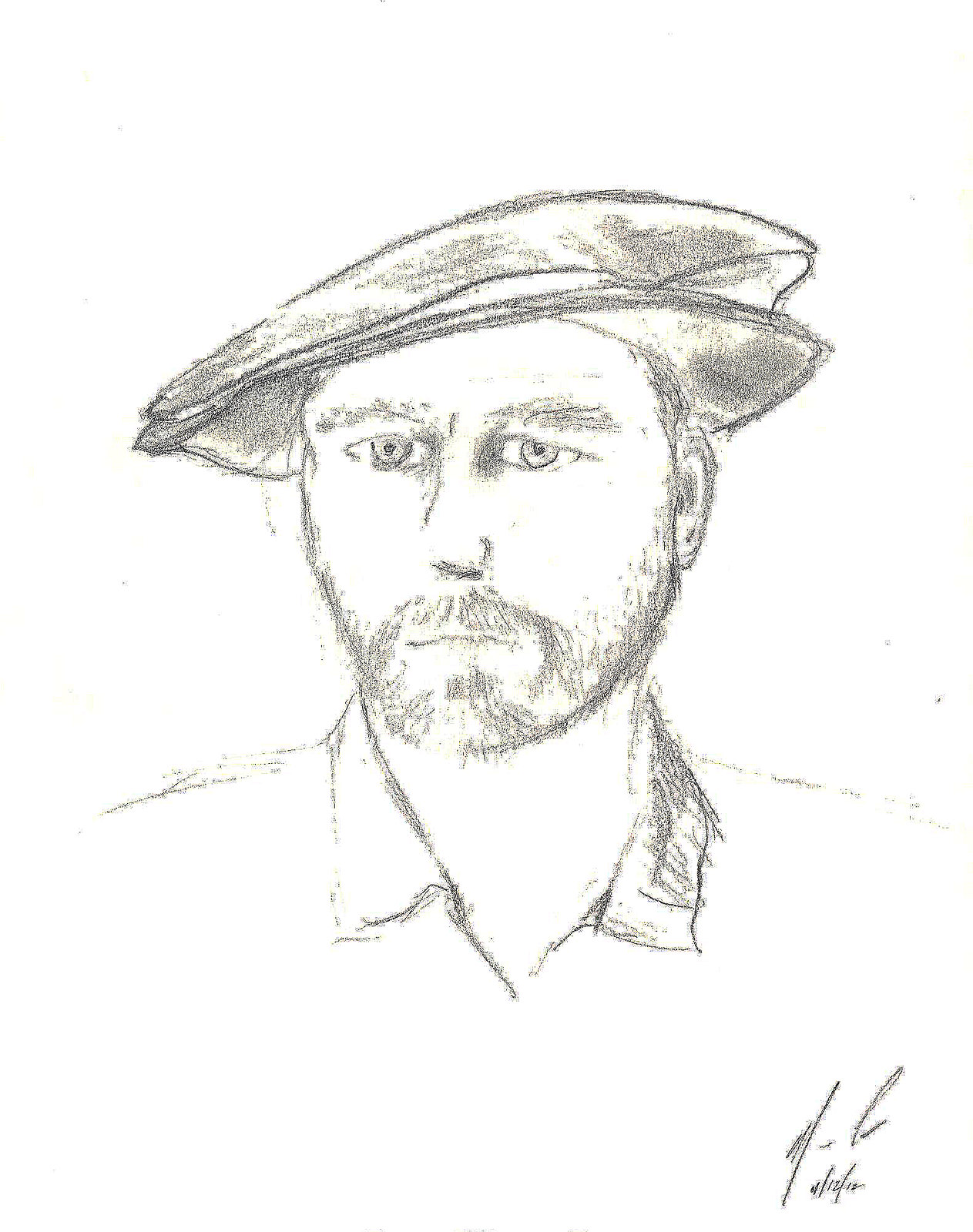This image is a pencil sketch on white paper, depicting a bearded man shown from the shoulders up. The drawing features a man with a rounder face, characterized by a closely trimmed beard forming a goatee, and thicker, heavy eyebrows. His left side is more prominently shown, exhibiting a slightly shaggy yet short hairstyle under an old-fashioned, beret-style hat, reminiscent of 16th or 17th-century headwear. The man's eyes are notably close together, and his facial features include a missing tip of the nose, leaving just the bridge and underpart drawn. He dons a collared shirt with bent-down collars and some shading on the left side. Despite the overall simplicity and light nature of the pencil line art, the image includes a signature and a date, possibly marked as 11-12-10, in the lower right-hand corner, though both remain indiscernible.